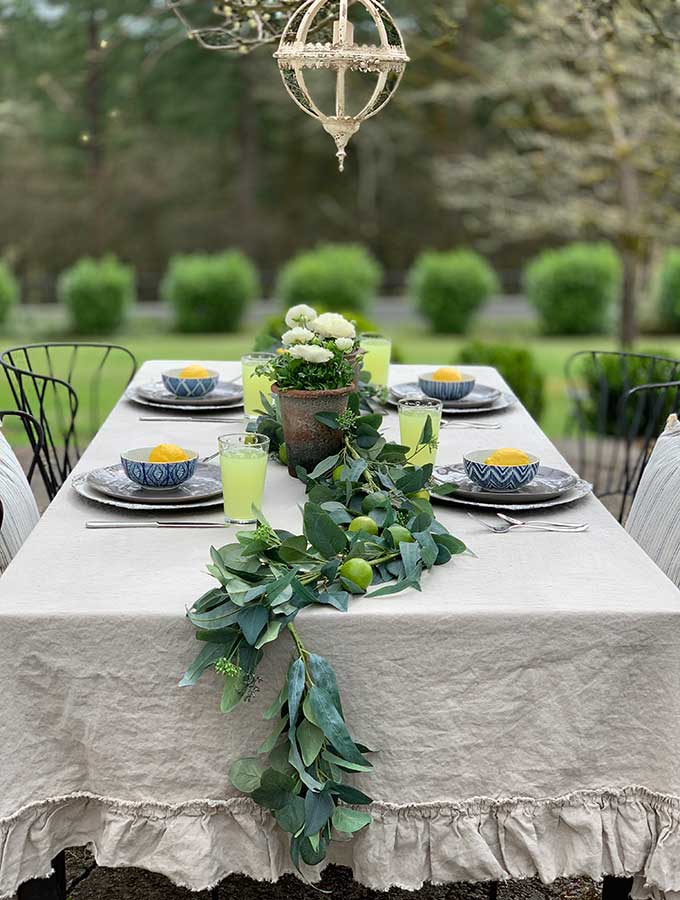In this image taken outside a home with a spacious yard, a meticulously set table stands as the focal point. The table, draped in a thick white tablecloth, features four place settings, each consisting of a base plate, an entree plate, and a bowl adorned with distinct blue and white patterns. Inside each bowl, an orange sherbet or ice cream adds a pop of color. There are also four glasses filled with a yellowish-green limeade. The center of the table is beautifully decorated with a flowerpot containing white flowers, flanked by green leafy vines and branches adorned with limes. Surrounding the table, well-trimmed bushes and a lush green lawn extend towards an out-of-focus backdrop that appears to be a forest. The scene evokes a sense of an elegant, possibly Victorian, outdoor brunch in a well-manicured garden.